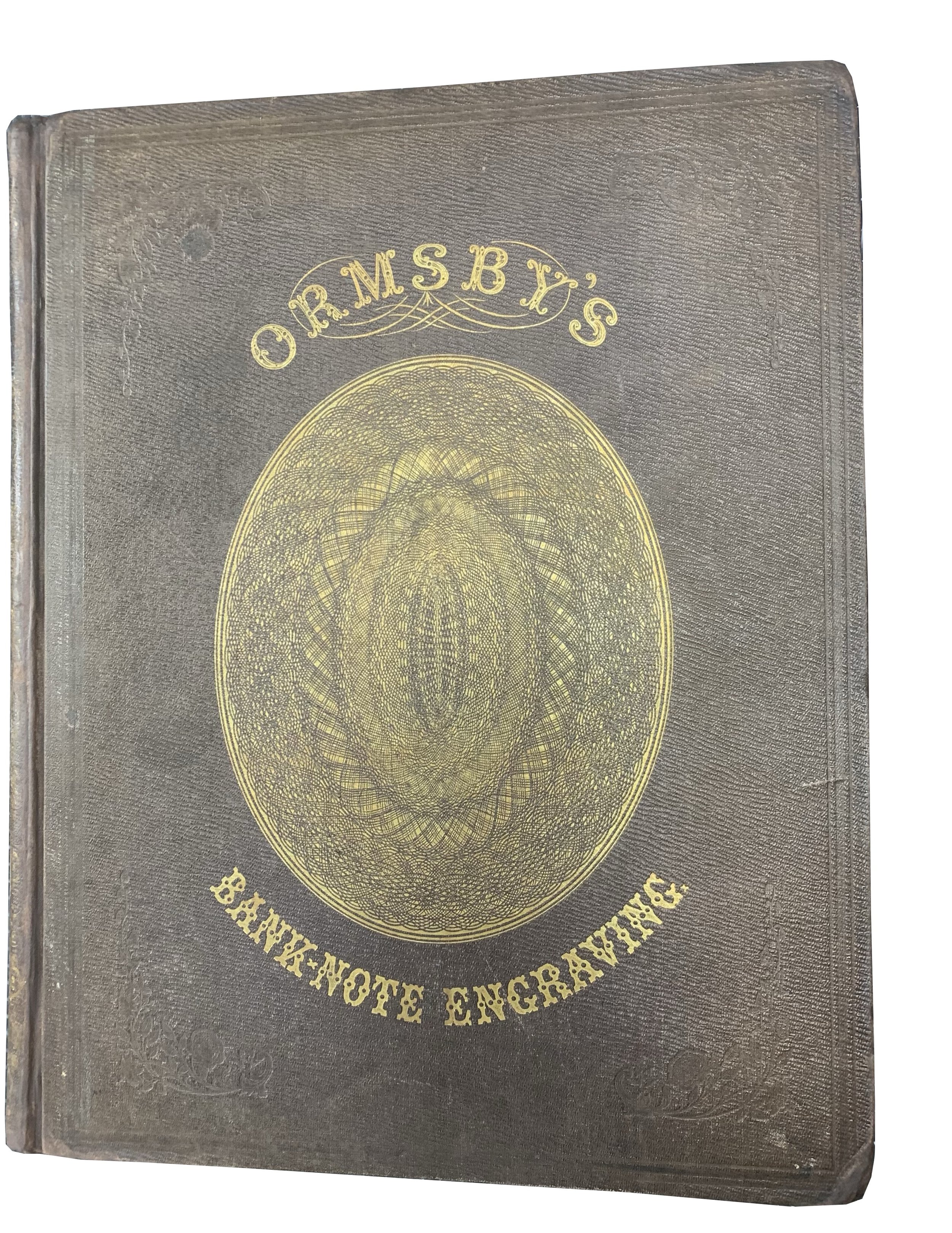The photograph features an antique, leather-bound book with a weathered, brown-gray cover. The book's texture suggests smooth, grained leather, with noticeable wear, including scratch marks and loose fibers along the binding. The cover is elegantly adorned with gold inlay, displaying a central oval design embellished with intricate patterns and a small floral motif at the bottom. Above the oval, the title "Ormsby's" is prominently displayed in ornate Gothic script, accompanied by decorative swooshes. Below the oval, the subtitle "Banknote Engraving" is written in the same gold Gothic text. The photograph is well-lit, showcasing the book's unique and historical aesthetic against a clean white background.